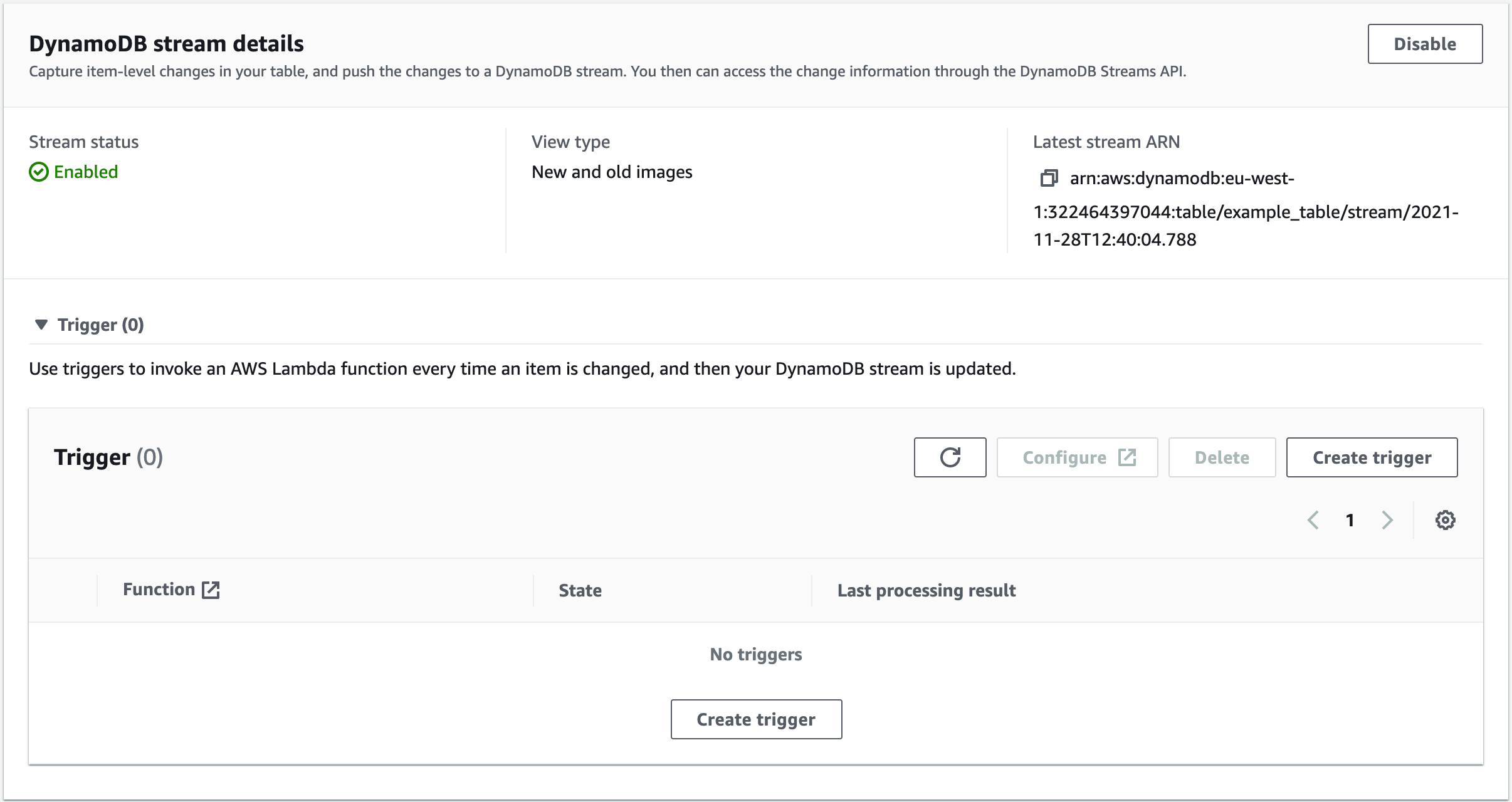This screenshot displays a highly technical dashboard tailored for IT professionals, specifically for managing Amazon Web Services (AWS) DynamoDB Streams. The interface boasts a clean, white background and offers detailed information regarding DynamoDB Streams.

At the top-left corner, "DynamoDB" is prominently featured in bold text, with "DB" capitalized, signifying it as a consolidated term. Directly below, the title reads "DynamoDB Stream Details" followed by a brief description: "Capture item level changes in your table and push the changes to a DynamoDB Stream. You can then access the change information through the DynamoDB Streams API."

In the top-right corner, there is a rectangular section, which appears to be disabled and is displayed in white. Returning to the left side, the "Stream Status" section shows a checkmark next to "Enabled," indicating that the stream is currently active.

Centrally, the "View Type" is specified as "New and Old Images," providing insights into the state of database items before and after changes. On the right side is the "Latest Stream ARN" followed by an extensive string of code, which is intentionally left unread for brevity.

Below this, a new section marked "Trigger" appears, including an inverted triangle icon, likely representing a dropdown menu. The accompanying text explains, "Use Triggers to Invoke an AWS Lambda Function Every Time an Item is Changed. Your DynamoDB Stream is updated."

This is followed by another headline labeled "Trigger," with a count of zero indicated. In the far-right corner, a gray outlined rectangle contains the text "Create Trigger," inviting users to set up new triggers for Lambda functions.

This detailed caption ensures that all critical information presented in the screenshot is conveyed comprehensively.